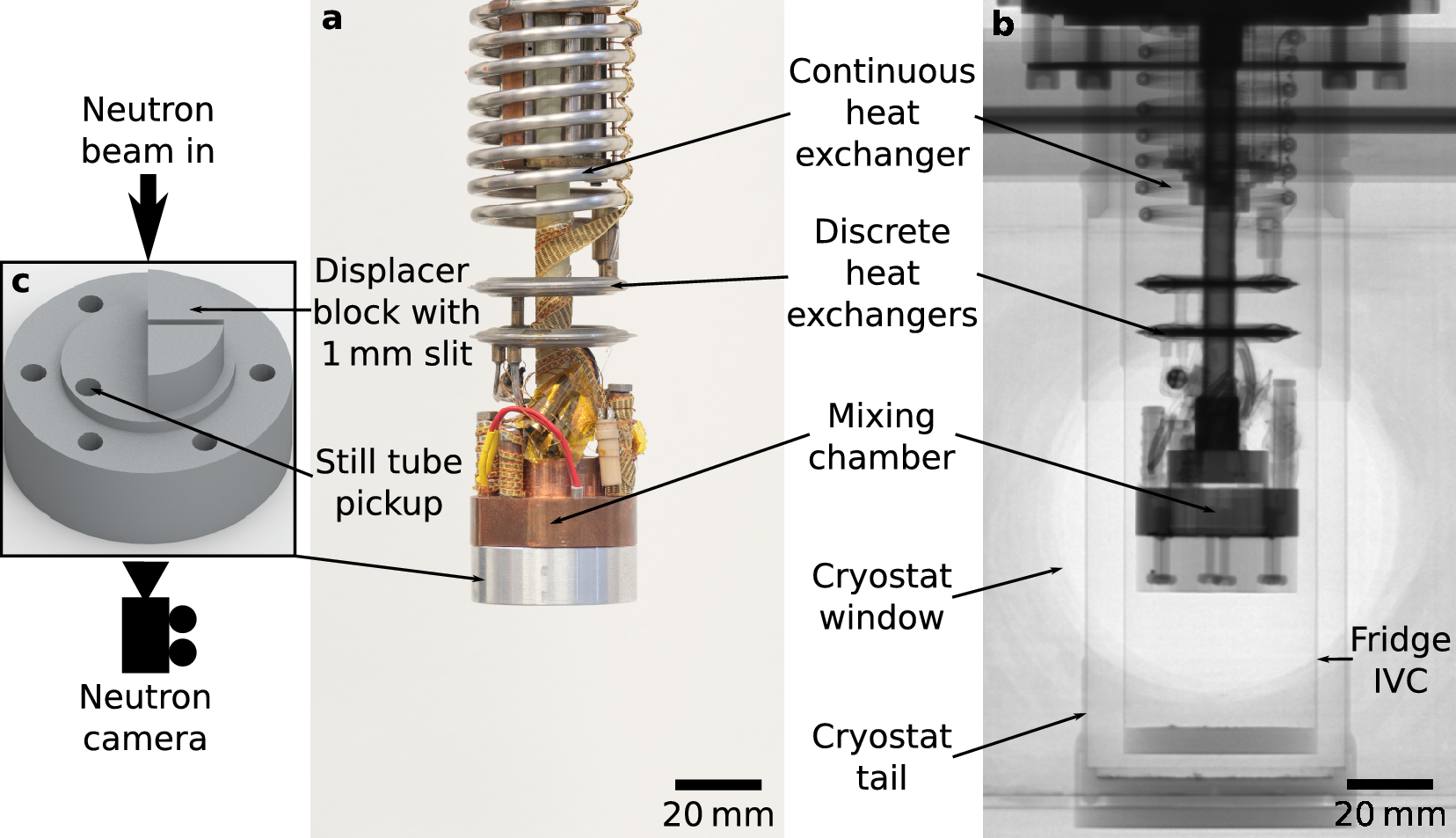The image is divided into two sections, depicting detailed diagrams of a mechanical device that resembles a piston or a complex heat exchanger system. 

On the left side, the image is annotated with various labels identifying specific components such as a "continuous heat exchanger," "discrete heat exchangers," a "mixing chamber," a "displacer block with a 1-millimeter slit," and an area marked "still to pick up." These labels provide a comprehensive breakdown of the device's internal mechanisms, highlighting how each part functions within the system.

The right side of the image presents a black-and-white version of the left diagram, giving it a stylistic appearance similar to a technical stamp or blueprint. This section also prominently displays a shock absorber-like component situated at the top of the piston. The bottom section of this diagram includes a measurement indicator, clearly reading "20 millimeters," which likely specifies the size of the device or a crucial dimension within the mechanism.

Overall, the combined images provide an intricate and highly detailed visual representation of the mechanical device, along with essential annotations and measurements for thorough understanding.